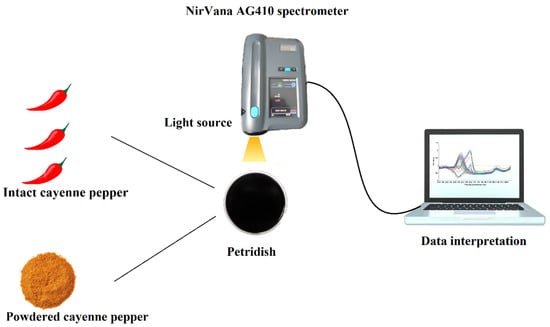The infographic image showcases the Nirvana AG-410 spectrometer. At the top, the title "Nirvana N-I-R-V-A-N-A AG-410 spectrometer" is prominently displayed. Below this, the spectrometer, a gray device with a small screen, is depicted. Attached to the spectrometer, and labeled as "light source," is a beam of light directed towards a black circle labeled "Petri dish." On the left side of the Petri dish, two arrows point towards images of cayenne peppers; one arrow, labeled "intact cayenne peppers," points upward towards three whole red peppers, while the other arrow, labeled "powdered cayenne pepper," points downward towards a pile of powdered pepper. To the right of the Petri dish, a cord connects the spectrometer to a laptop displaying a graph, with the label "data interpretation." This detailed diagram illustrates the process of analyzing both whole and powdered cayenne peppers using the spectrometer's light source and data interpretation capabilities.